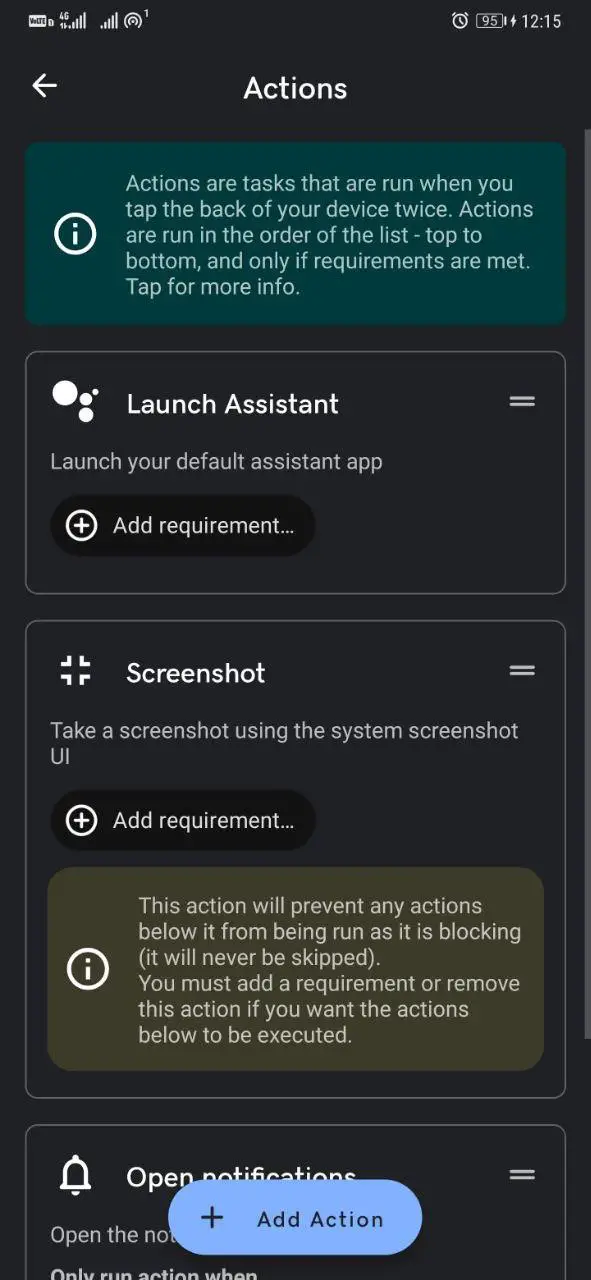This is a detailed screenshot taken from a mobile phone, showcasing its interface. At the top, there are several status icons: a full Wi-Fi signal, full mobile data signal, and a battery at 95% currently charging. The time displayed is 12:15.

Below the status bar, a dark blue window is open, with "Actions" written in white font at the top, accompanied by a small arrow pointing to the left. Directly beneath this, there's a lighter blue rectangle featuring an icon of a white "i" encircled, followed by the text: "Actions are tasks that are run when you tap the back of your device twice. Actions are run in the order of the list top to bottom and only if requirements are met. Tap for more info."

Following this explanation, there is a grey rectangle labeled "Launch Assistant," which allows launching the default assistant app. Underneath, a black oval with the text "Add Requirement" in white font features a plus sign (+).

Next, there is a white rectangle with the text "Screenshot," which facilitates taking a screenshot using the system’s screenshot UI. Similarly, below this is another black oval with "Add Requirement" in white font, also incorporating a plus sign (+).

At the bottom of the window, there is a red box containing a small white circle with an "i" in the center, indicating additional information.